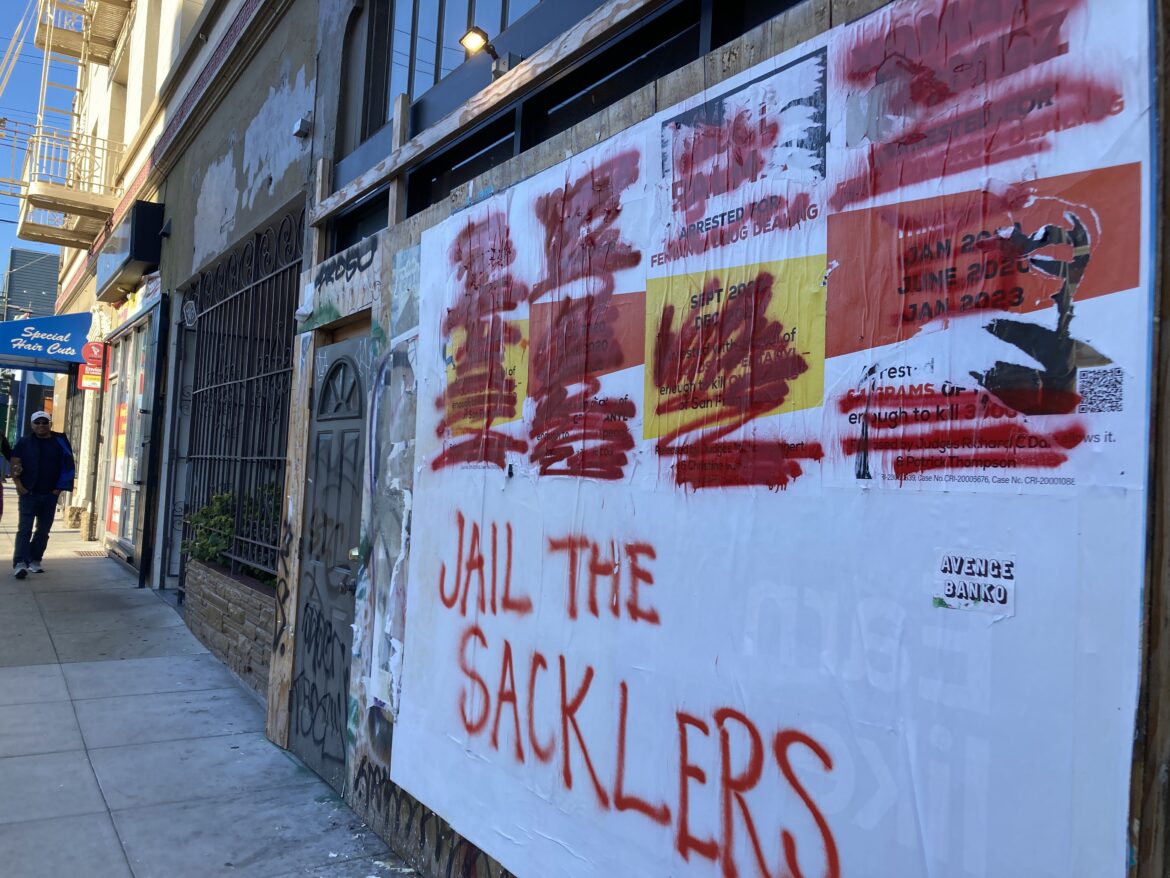The image captures a gritty urban scene in a bustling city. Central to the photograph is a decaying, boarded-up building with a white tarp covering part of it. The tarp is heavily defaced with red graffiti that reads "Jail the Sacklers," a reference to the controversial Sackler family associated with Purdue Pharma. The graffiti also obscures an image underneath, with additional markings crossing it out. To the right, there's an unobstructed QR code on the tarp. Below the red text is another tag, "Avensi Banco," though its meaning is unclear.

The foreground reveals a sidewalk and a street scene at an angle, with a pedestrian walking towards the camera. The person is dressed in a black jacket, white hat, and dark pants. To the left, a blue sign bearing the partially legible name "Special Something Cafe" is mounted on a building with a visible fire escape. Black bars or gates frame parts of the structure on the right side. The photo also captures a bit of the surrounding area, suggesting a cityscape of neglected infrastructure and spontaneous urban art.